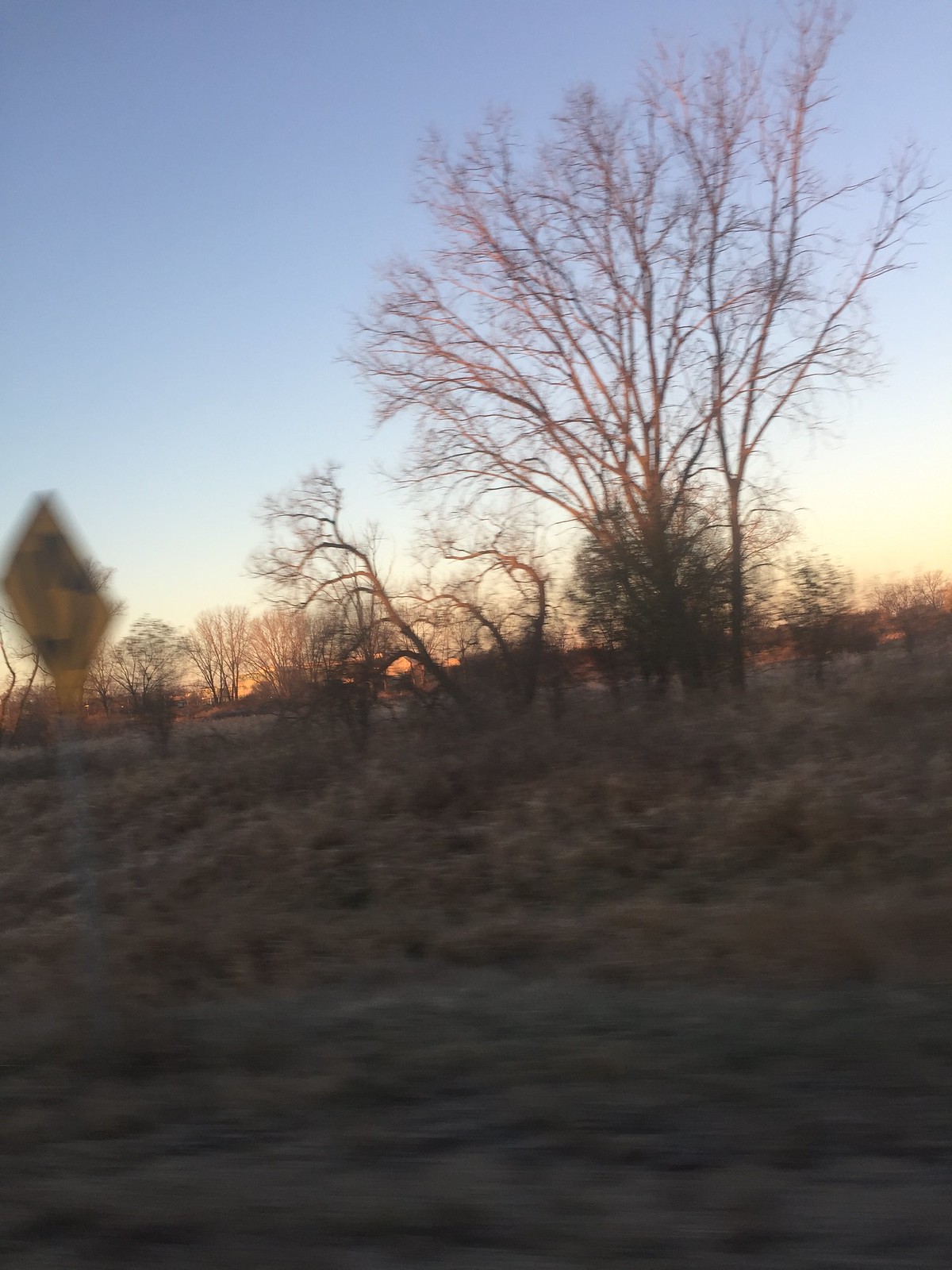The photograph is a color image capturing a rural landscape during sunset. The top half of the image is dominated by a gradient sky, transitioning from a deep blue at the top to a pink-orange hue near the horizon, indicative of the setting sun. The bottom half is characterized by a patchwork of grayish dirt and dry, brushy grass, suggesting a very arid environment. The foreground appears slightly blurred, possibly due to the photo being taken from a moving vehicle. 

In the middle ground, there are several dormant trees devoid of leaves, with their branches stark against the evening sky. Among these, larger trees occupy the center-right portion of the image, extending across the sky. Sparse bushes also intermingle with the trees. 

A notable feature on the left side of the image is a blurry, diamond-shaped yellow street sign, adding a touch of human element to the otherwise nature-dominated scene. The overall setting looks tranquil and undeveloped, with no visible traces of urban development, amplifying the rustic and serene nature of the landscape.